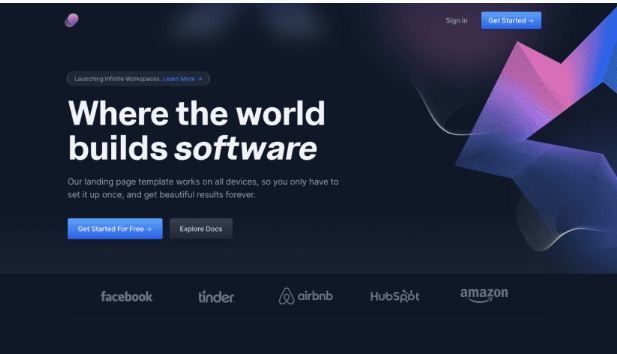The home page of the unidentified company features a sleek black background adorned with striking purple and blue geometric patterns on the right side. The top navigation bar includes options to "Sign In" or to "Get Started," which prompts users to register. The page appears to offer templates for various services and devices, potentially for building custom web pages. The prominent header reads, "Where the World Builds Software," emphasizing that their landing page template is compatible with all devices, offering a one-time setup that ensures aesthetically pleasing results indefinitely.

Highlighted in blue, there are primary call-to-action buttons: "Get Started for Free" and "Explore Docs." Below the main header, a section showcases well-known websites that presumably utilize this service, including Facebook, Tinder, Airbnb, HubSpot, and Amazon. A small, purple circular icon is positioned at the top left corner, adding a subtle yet noticeable branding element. The overall design is modern and user-friendly, encouraging ease of access and engagement.